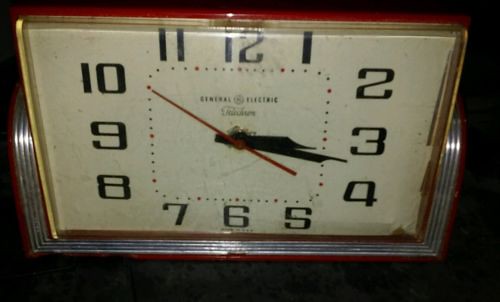This is a color photograph showcasing a close-up view of an antique clock face, observed from a top-down angle. The clock, with a square or slightly rectangular structure, exudes vintage charm. The bottom of the clock features a dark area, accentuated with a slender red rim and an inner gold rim that gleams under the light, giving parts of it a silvery appearance. Encircling the clock face are black numerals arranged in a square format, marking the hours from 1 to 12. Positioned at just past a quarter past three, the clock's black hour and minute hands are prominently displayed, along with a thin red second hand pointing to the 10-second mark. Central to the clock and slightly above the hands is a delicate black logo and some joint-up writing, too small to discern clearly. The clock face is subtly illuminated, with light reflections noticeable especially around the edges, bottom, and just above the 12 o'clock position.